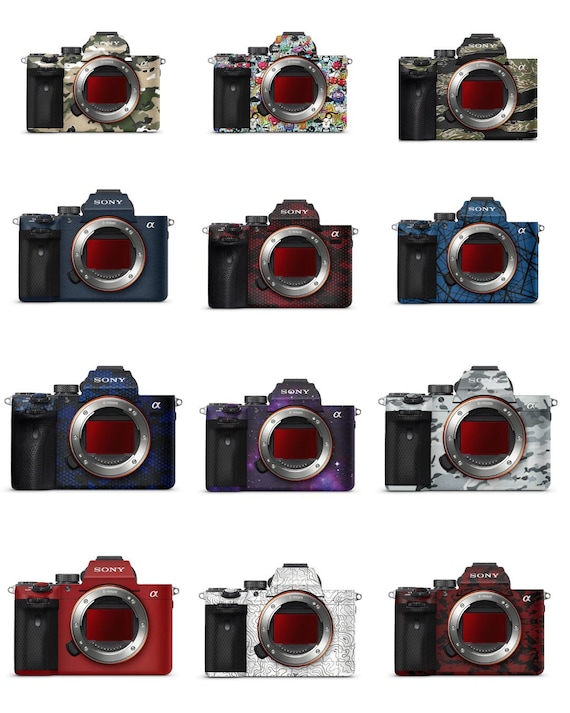This image features a meticulously arranged collection of twelve vintage Sony manual cameras, each adorned with a unique skin or design. The cameras are organized into four vertical columns and three horizontal rows against a pristine white background, creating the illusion that they are floating midair. Each camera prominently displays the Sony logo and features a circular lens with a silver ring. The top row includes a camouflage design, a colorful cartoon collage, and a map-like pattern. The second row showcases a monochrome blue camera, a red and black lava-like design, and a predominantly blue camera with diagonal black lines. In the third row, there's a dark blue camera with a sheen, a purple one with white stars resembling a night sky, and an urban camo design. The fourth row features a solid red camera, a white camera with rounded gray squiggly lines, and another red and black lava-like patterned camera. Despite their differing appearances, all cameras share nearly identical design attributes, giving the image a structured and cohesive look as part of what appears to be an advertisement.